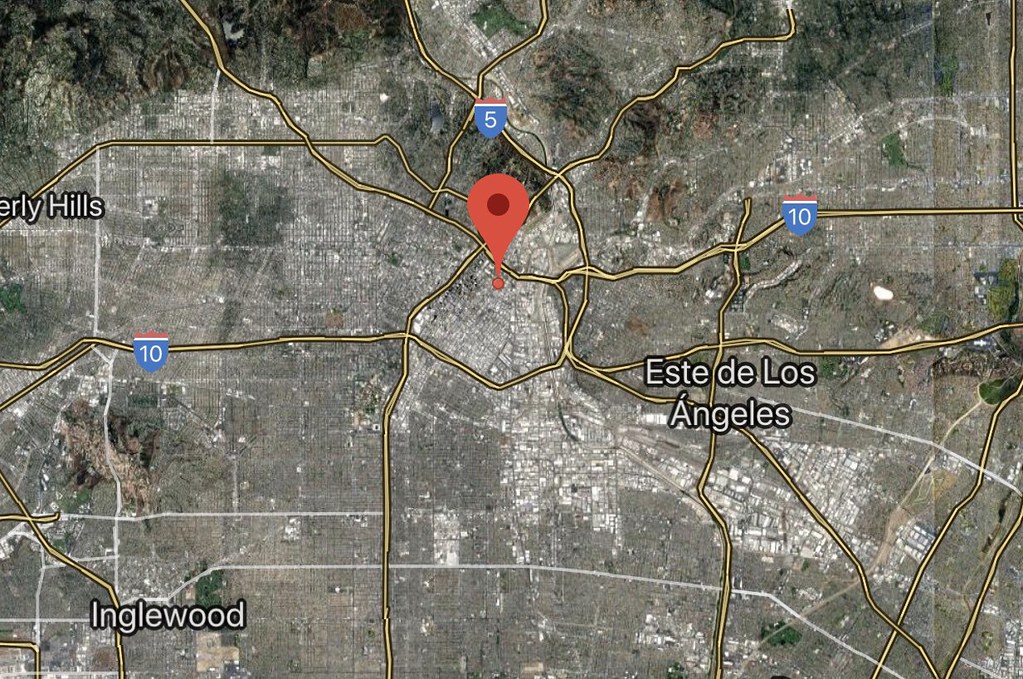This aerial view appears to be a map, possibly sourced from Google Maps or Apple Maps. The landmass is depicted in varying shades, with densely populated areas appearing in a grayish color, transitioning to a lighter gray mixed with white. Vegetation such as grass and trees are shown in green and brown hues, while the roads are marked in an orangish-yellow color with black borders.

The topography features three prominent hills. One hill enters from the left side about two inches from the top and extends rightward just shy of the image's center before continuing upward off the screen. Another hill appears approximately an inch in from the right corner and descends slightly before going off the top of the page. A third hill emerges in the right center, about half an inch in from the edge, extending downward for about an inch before leaving the frame. The remaining terrain is predominantly brown with scattered hilly regions.

The map details several roads: four roads extend from the top, with one on the far left, two towards the middle, and one on the far right. Additional roads come in from various sides, creating a clustered intersection in the map's center.

Key landmarks and text include:
- The letters "E-R-L-Y" near the hills in the top left corner.
- "Englewood" in white lettering positioned just right of the bottom left corner.
- "Este De Los" and "Angeles" near the center-right, with "Este De Los" situated above "Angeles".
- A freeway sign with a white "10" inside a primarily blue shield, located near the center-right. An identical sign appears around three inches up and to the left, and another "10" sign is almost in the center, about two inches from the left.
- A similar freeway sign with a white "5" is placed about three inches to the left and up from the first "10" sign.

Prominently in the map's center is a large red pin, indicating a specific location, with the center of the pin being a darker red.